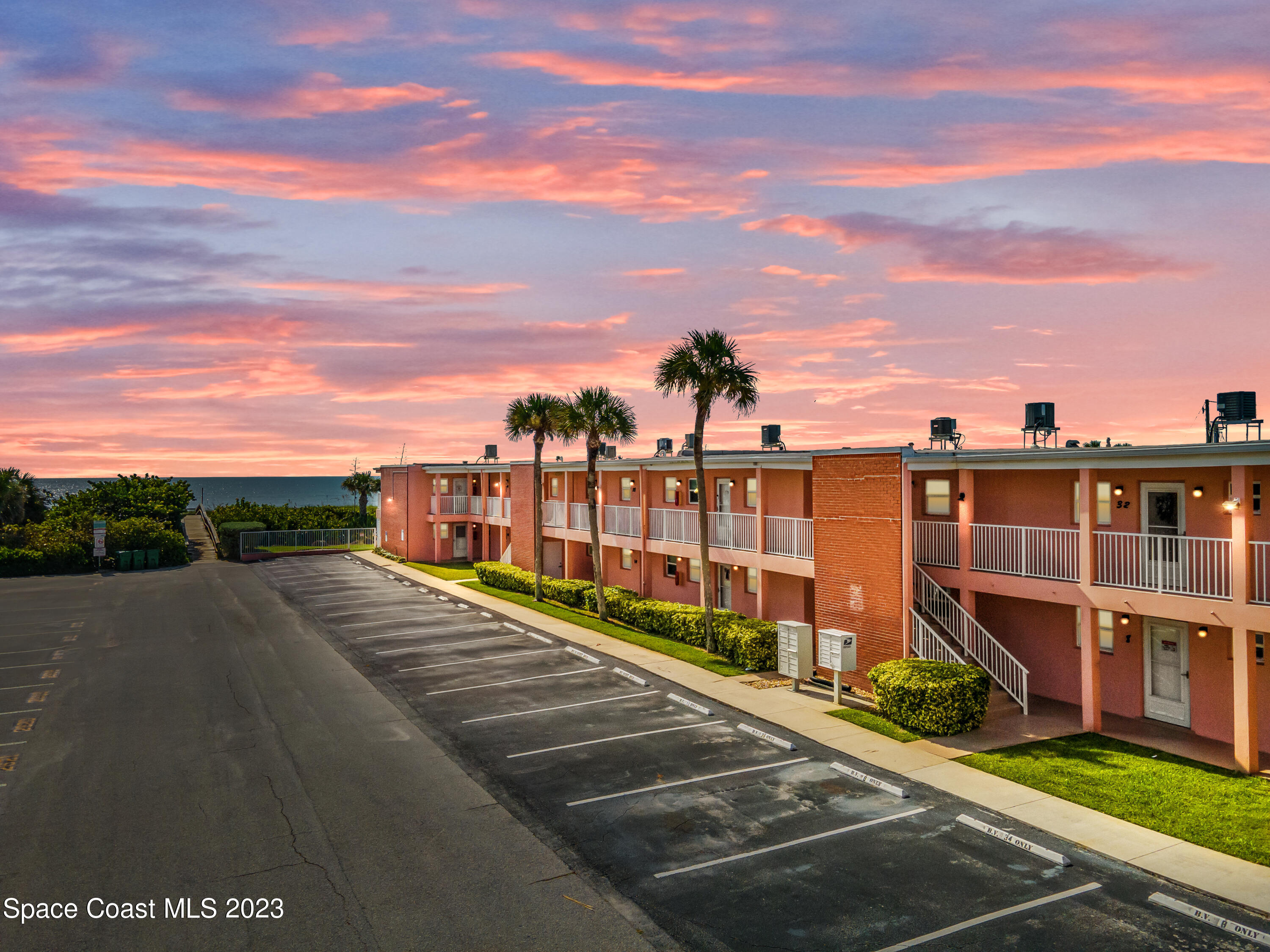This image captures a long, two-story building reminiscent of a coastal town motel. The structure features numerous doors on both the ground and upper levels, each accompanied by a small window. The upper story is accentuated by thin balconies with metal railings running across its length. The building is painted orange and flanked by lush hedges and palm trees, further hinting at its seaside location. In front, an extensive asphalt parking lot, demarcated with white lines and equipped with parking bumpers, sits empty. Viewing this scene at dawn, the sky is adorned with a blend of orangey, pink, and blue hues, with streaks across the clouds, and the horizon reveals a shimmering expanse of aquamarine ocean waters. In the background, a row of low shrubs and bushes adds depth to the setting, enhancing the coastal ambiance. White text on the bottom left corner of the image reads "Space Coast MLS 2023," suggesting its relevance to a real estate multi-listing service.